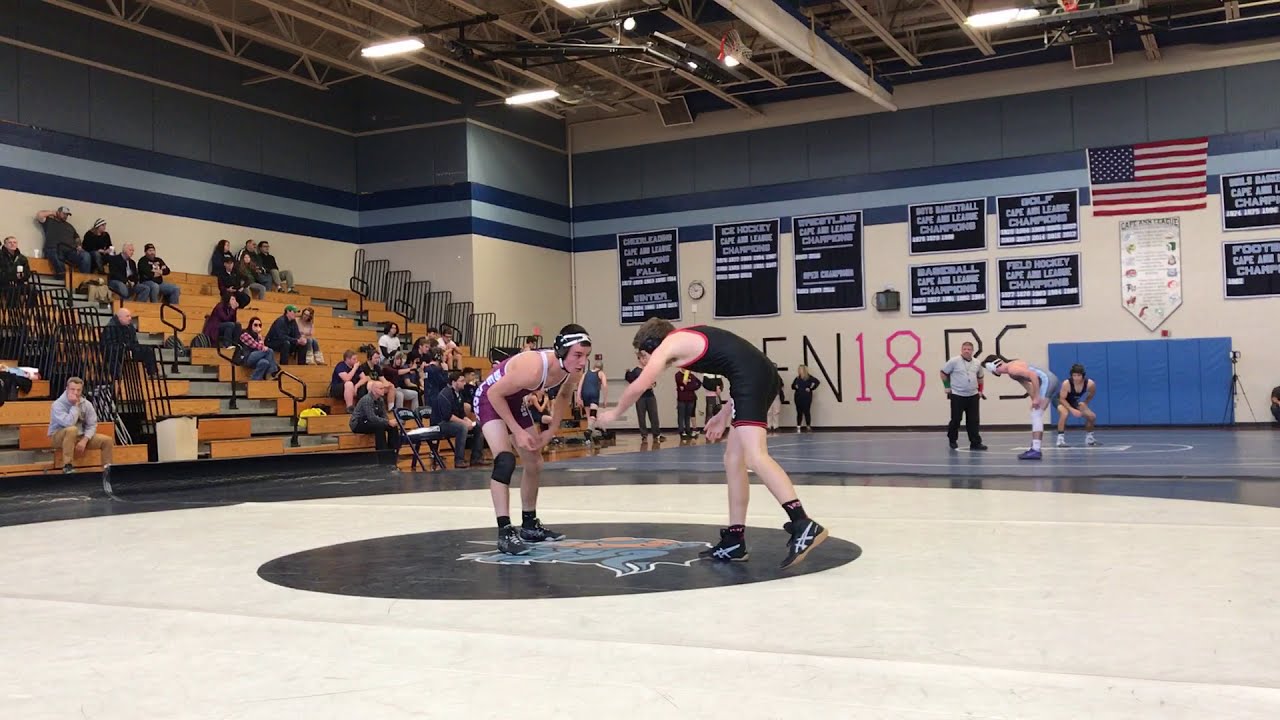This detailed photograph captures an intense moment at a school gymnasium during a wrestling tournament, where two boys, dressed in wrestling uniforms, are about to engage in a match. The wrestler on the left is clad in a maroon and white uniform, equipped with protective headgear and a single knee pad. His opponent wears a black and red uniform with black and white shoes. They are positioned at the center of the gymnasium floor, standing on a large black symbol on a tan surface. Both wrestlers are hunched forward, eyeing each other with focused determination.

The gymnasium's walls are painted in light blue, dark blue, gray, and tan, providing a vibrant backdrop. Above the wrestlers, a lighting setup illuminates the scene, casting defined shadows. To the left, spectators are seated in stadium bleachers, closely watching the match unfold. The back wall features an American flag and several banners, with the letters and numbers "FN18BS" prominently displayed. Additionally, a blue mat is seen near the posters and flag. Not far behind the central wrestlers, another pair of competitors is seen preparing for their bout, adding to the dynamic and lively atmosphere of the athletic event.